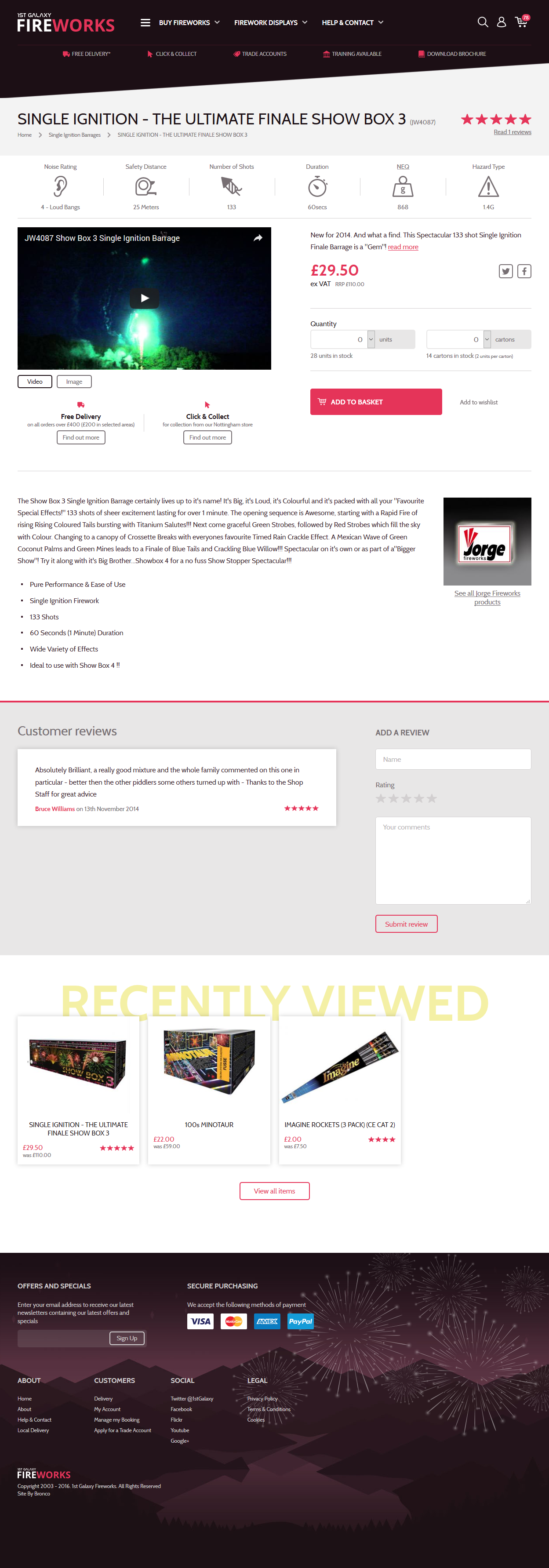Here is a cleaned up and detailed descriptive caption for the screenshot you described:

---

The screenshot, though initially barely legible, reveals considerable detail upon magnification. Positioned at the top is a black header where the word "Fireworks" is prominently displayed in white font. This header features several more options in a similar white font, accompanied by tabs in a smaller white sizing.

Underneath this header, the text "Single Ignition The Ultimate Finale Showbox" with a five-star rating is clearly visible. Adjacent to this, there is an image depicting a green explosion confined within a black rectangle. The price listed for this exclusive item is £29.50.

Beneath the image and the pricing, a red bar is present, followed by a comprehensive paragraph that elaborates on the product, offering an exhaustive checklist of features.

On the far right of this descriptive paragraph, there is an icon seemingly labeled "George" with a "J," situated above a gray rectangle that introduces the section "Customer Reviews." This section includes a sample review and a text box provided for users to submit their own feedback.

Just below the "Customer Reviews" section, a "Recently Viewed" area showcases three different products that a user has recently examined.

Finally, the footer of the screenshot features a photo-infused background portraying a purplish mountain range. This area includes logos of major credit cards interspersed with white text. At the very bottom, the word "Fireworks" is reiterated.

---

This caption should provide a clear and comprehensive overview of the details available in the screenshot.